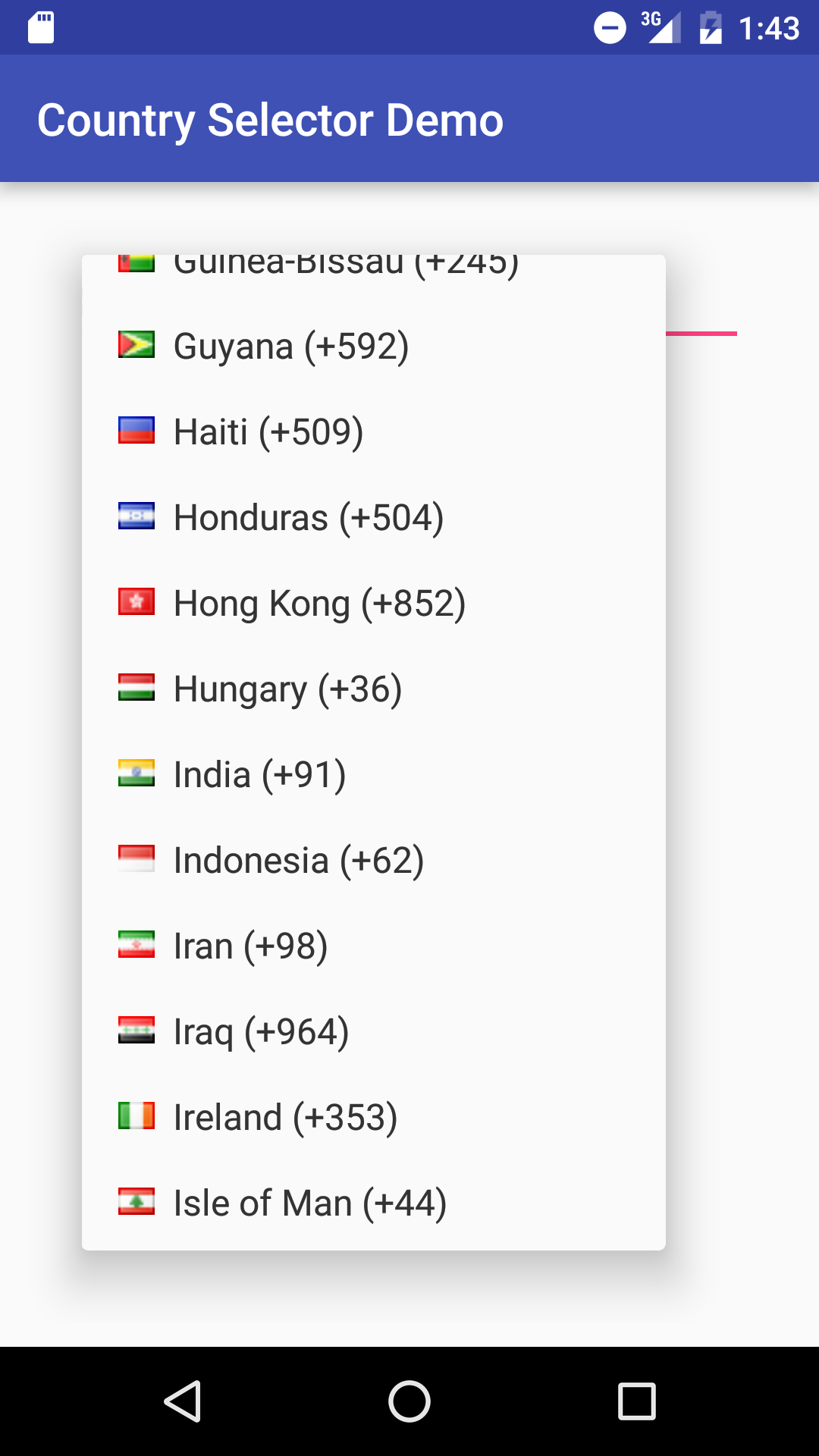Screenshot of a country selection drop-down menu titled "Country Selector Demo." The menu displays a pop-up window listing various countries and their corresponding international dialing codes. The countries are organized alphabetically and start with "Guinea-Bissau (+245)," followed by "Guyana (+552)" or possibly "Ghana (+552)." Other countries listed include "Haiti (+501)," "Honduras (+504)," "Hong Kong (+852)," "Hungary (+36)," "India (+91)," "Indonesia (+62)," "Iran (+98)," "Iraq (+964)," "Ireland (+353)," and finally "Isle of Man (+44)."